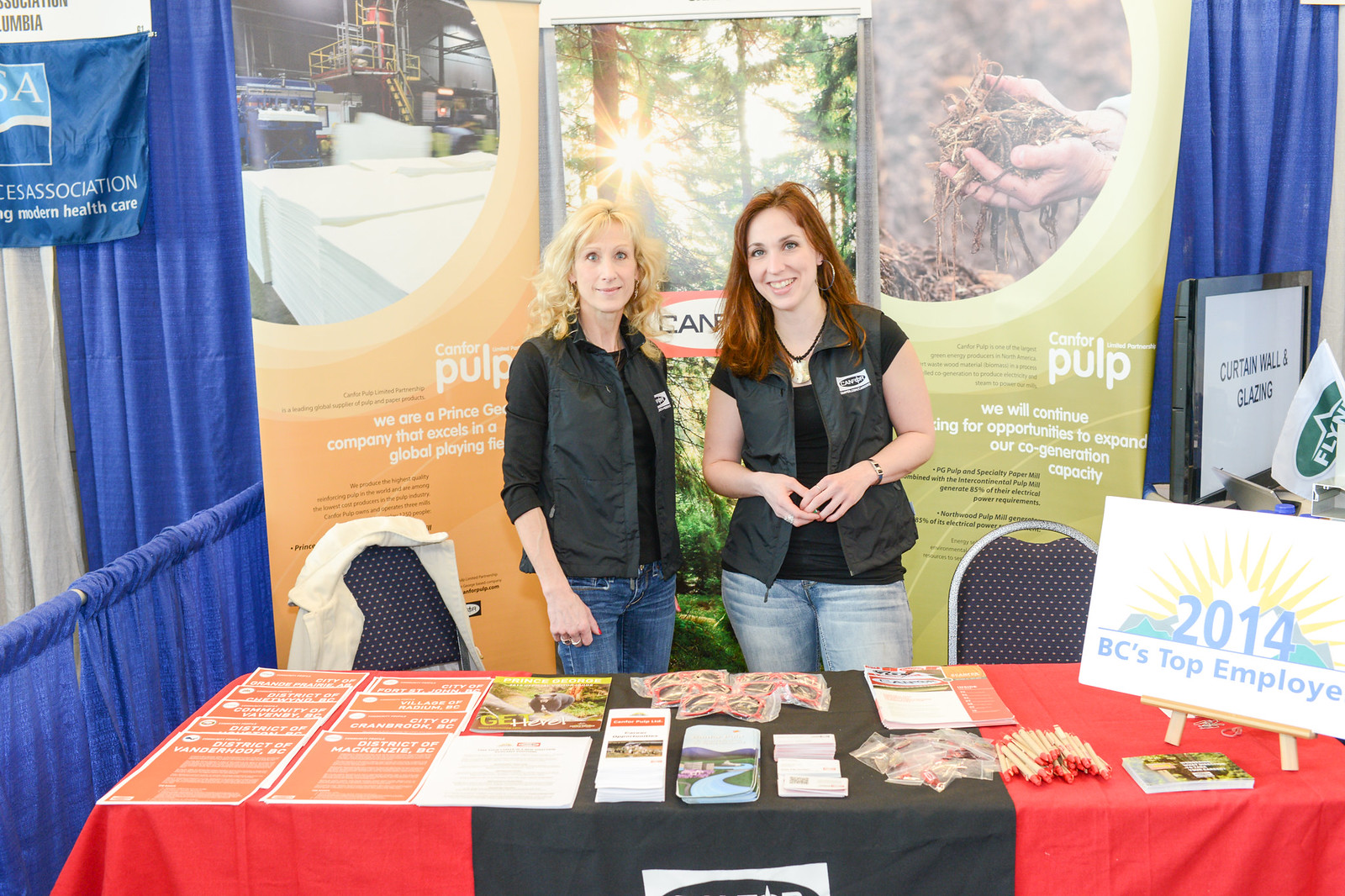The image showcases a vibrant booth at a convention, featuring two women standing behind a table covered with a red and black tablecloth. The table is laden with various promotional materials, including posters, pamphlets, buttons, and pens. Prominently placed to the right is a sign that reads "2014 BC's Top Employee," adorned with an illustration of a sun. The backdrop features banners depicting industrial scenes; the left banner illustrates a paper plant, while the middle one displays a forest landscape with a sunrise, and the right one shows hands digging into soil, emphasizing a connection to nature and sustainability. The two women, both wearing dark gray vests emblazoned with a company logo, smile warmly for the camera. The woman on the left has blonde hair, is slightly older, and is dressed in a black long-sleeve shirt and blue jeans. The woman on the right has auburn hair, appears younger, and wears a black short-sleeve shirt with light blue jeans. The booth represents a company involved in the paper industry, likely specializing in wood pulp and paper products. Adjacent booths are visible, and the natural quality of the lighting suggests the event could be outdoors, though it remains uncertain.